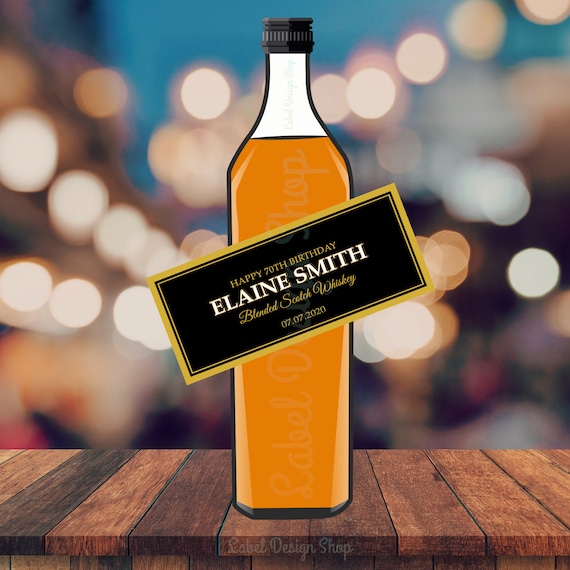This image presents a computer-generated, cartoon-like depiction of a bottle of blended scotch whiskey. The bottle features a sleek, tall design with a black twist-off cap and is filled nearly to the top with an orange-colored liquid. Prominently displayed on the bottle is a rectangular label that reads "Happy 70th Birthday Elaine Smith," with additional small text indicating "Blended Scotch Whiskey" and the date "07.07.2020." The bottle rests on a thin, uniquely patterned wooden table or railing. The background is blurred, adorned with numerous out-of-focus lights, giving the image a festive and celebratory ambiance.